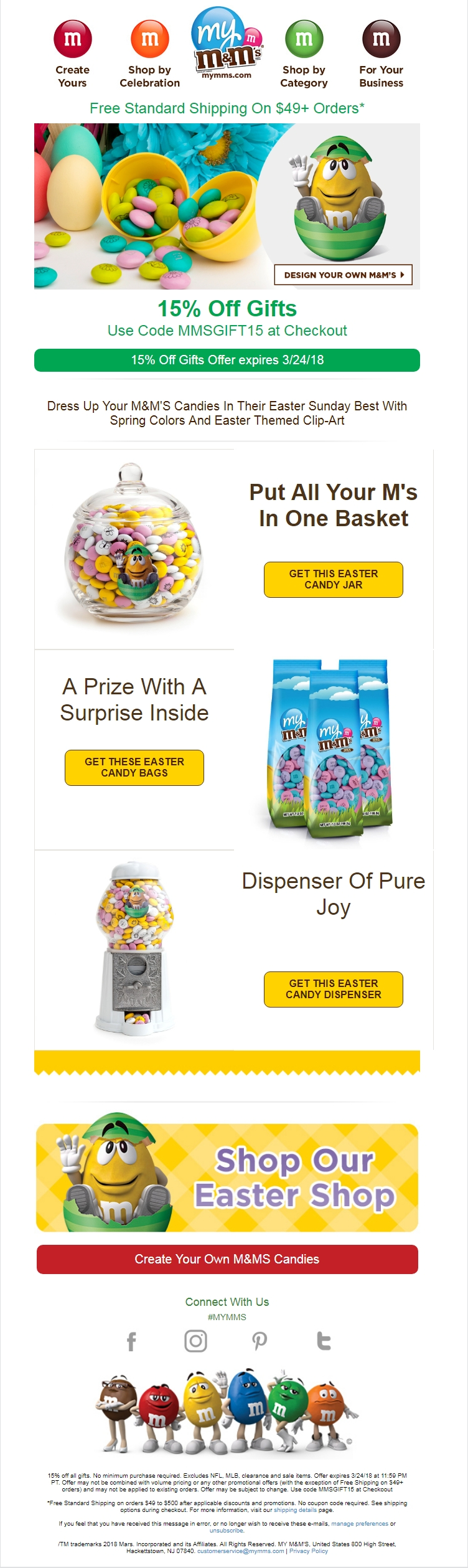The screenshot captures the homepage of the MyMMS.com website, elaborately adorned with various M&M-themed icons and banners. At the top of the page, a series of animated M&M characters traverse from left to right. The sequence begins with a red M&M above the text "Create Yours," followed by an orange M&M next to "Shop by Celebration." Adjacent to these is a large blue M&M beneath the website's name, "MyMMS.com." Continuing right, a green M&M labeled "Shop by Category" is next, followed by a brown M&M with the text "For Your Business."

Beneath this row of colorful characters, a prominent banner announces "Free Standard Shipping on $49+ orders." On the left side of this banner, there is an image featuring Easter-themed M&M's in a pastel color palette. Additionally, the iconic yellow peanut M&M character is whimsically situated inside a broken watermelon. Accompanying this character, the text reads "Design Your Own M&M's."

At the very bottom of the page, there is a footer highlighted with a vibrant purple text saying "Shop Our Easter Shop," set against a contrasting yellow background.